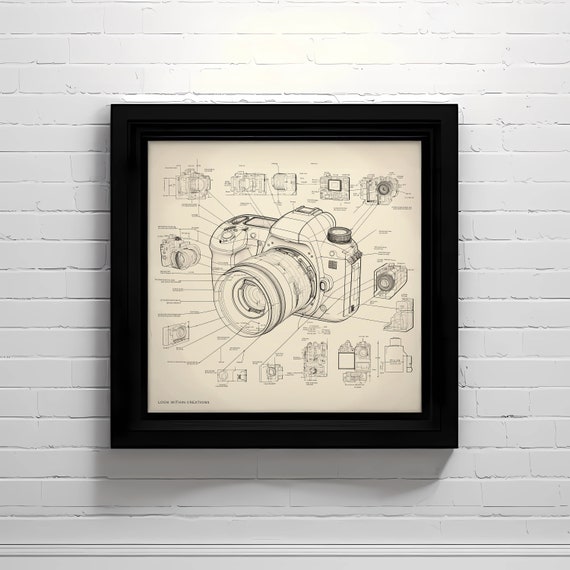This photograph captures a detailed framed illustration of a 35mm SLR camera, prominently displayed against a white brick wall. The artwork, rendered in black pen and ink on pale yellow paper, is encased in a simple, square black frame that measures a few inches wide. The camera illustration is positioned at a slight 30-degree angle to the left and features meticulously labeled components, including various knobs and buttons. Lines extend from the main camera image to smaller, detailed drawings of each part, offering a close-up view of the intricate mechanisms. Although the labels and words near the bottom left corner of the illustration remain illegible, the depiction of the slightly extended lens barrel, subject to detailed annotations, highlights the complexity and precision of the artwork.